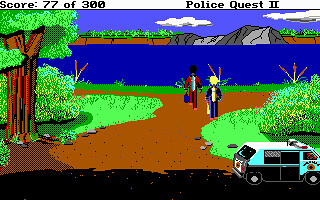The image appears to be a screenshot from the video game "Police Quest 2." The scene is vibrant and teeming with life, showcasing tall trees and lush green grass that blanket the area. In the lower right corner, a black and white police cruiser SUV is prominently positioned, complete with operational police lights on its roof. Two men are seen approaching the cruiser; one is dressed in red, while the other is in blue. In the background, there is a hint of water and the distant silhouettes of mountain tops, adding depth to the picturesque environment. The top of the screen displays the game’s score, indicating 77 out of 300 points, and prominently features the game's title, "Police Quest 2," on the right-hand side.